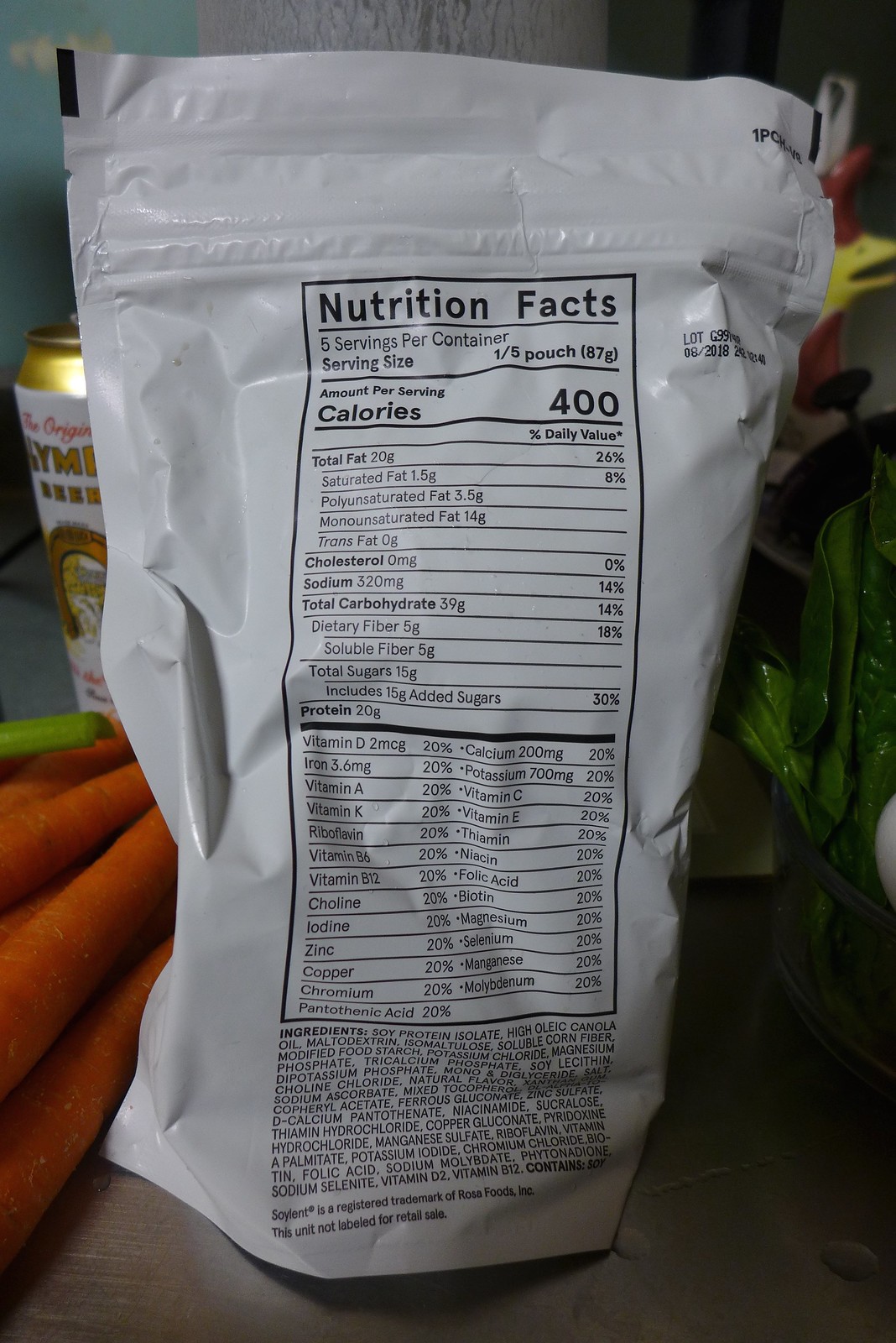This is a detailed photograph of the back of a white plastic bag, likely a chip or food product bag, sitting on a brown table. The bag features a distinct black rectangular section displaying the nutrition facts which indicate the product contains five servings per container, with a serving size denoted as one-fifth to one-sixth of a pouch and each serving containing 400 calories. Additional nutritional information such as total fats, cholesterol, sodium, total carbohydrates, and proteins are meticulously listed. At the very bottom of this section, the bag displays a list of ingredients and also mentions that "Soylent" is a registered trademark of the production company, adding that this unit is "not for retail sale". 

The scene also includes several items on the table: a bundle of orange carrots with a piece of celery laid on top of them, situated to the left of the bag. Adjacent to the vegetables is a beer can or canned beverage with a gold top and a white label, partially obscured by the bag. The background showcases a powder blue wall in the top left corner, transitioning to a white wall with visible cracks in the top center. Additionally, a bowl or basket filled with green leaves is visible in the bottom right corner of the image.